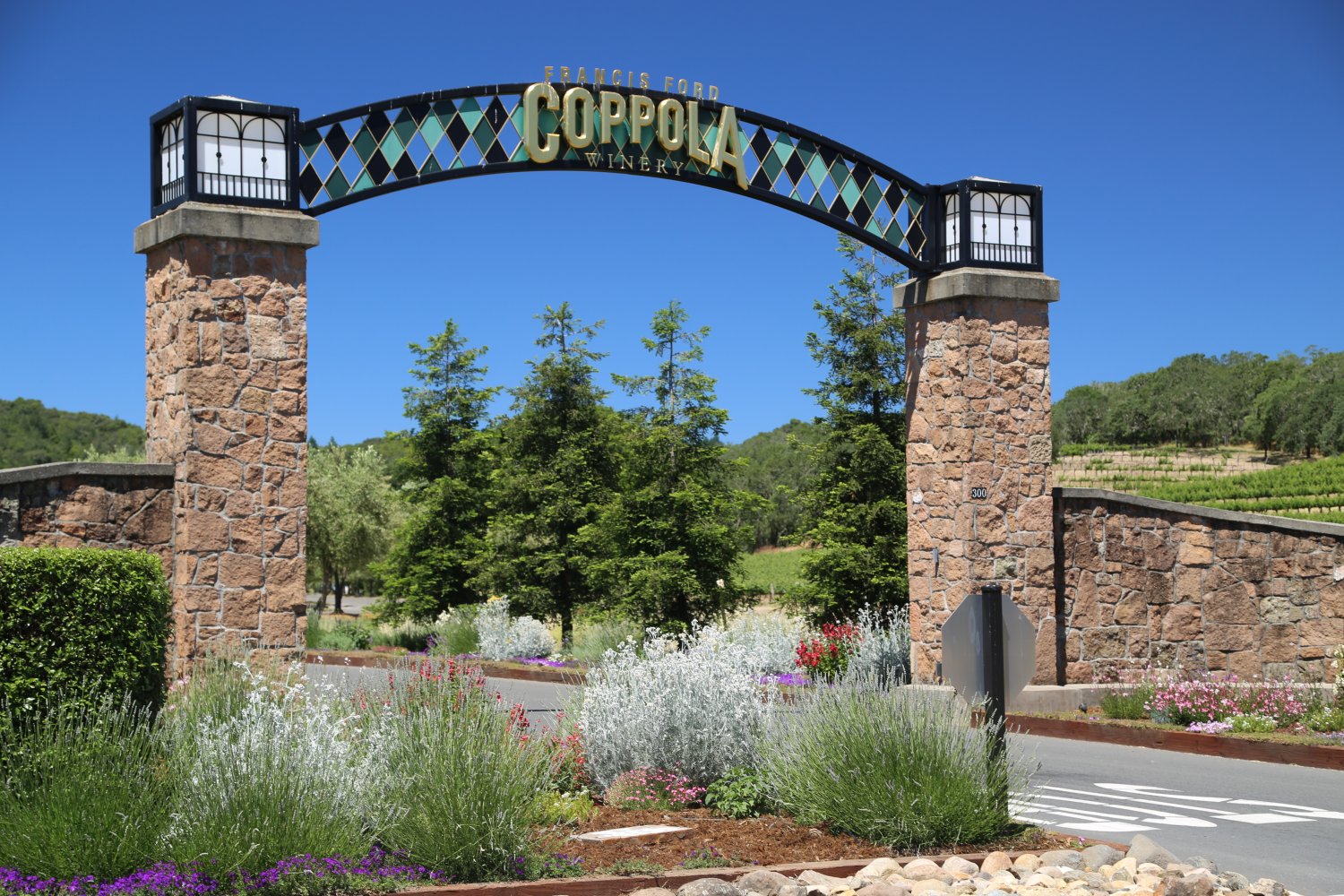The image features the grand entrance to the Francis Ford Coppola Winery, marked by two robust stone pillars topped with concrete. The pillars support an elegant archway adorned with diamond-shaped stained glass sections in varying shades of blue and green, outlined in black. Centered on the arch, the winery's name is proudly displayed in gold lettering, with "Coppola" in the largest letters.

At the base of the pillars, meticulously landscaped flower beds feature lush green shrubs, some with red leaves, and other plantings, including thin, straight-leaved bushes and some flowers with purple ends. The entrance leads into a narrow roadway, barely visible behind the dense foliage, which has white lettering on it.

In the background, tall pine trees rise majestically against a flawless, cloudless blue sky. To the right, rolling hills are lined with neatly arranged grapevines, emphasizing the vineyard setting. The overall scene is serene and inviting, capturing the essence of the winery's elegance and natural beauty.